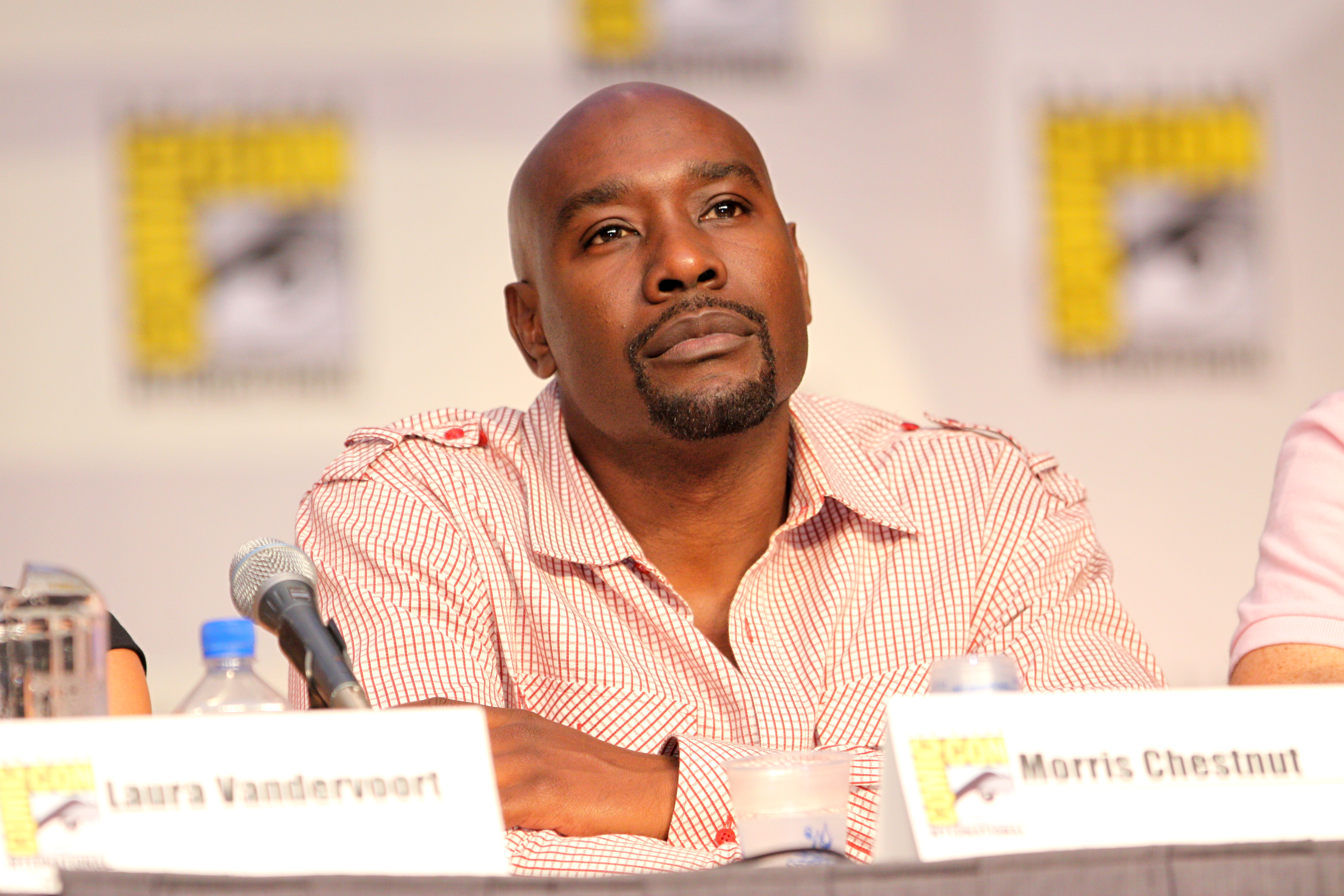The photograph captures Morris Chestnut, an African-American actor, at San Diego Comic-Con. He is seated at a table, wearing a distinctive long-sleeved, collared shirt with a white and red checkered pattern. Morris has a shaved head and a neatly trimmed goatee. In front of him, a nameplate clearly displays his name. To his left, another nameplate reads "Laura Vandervoort." The background prominently features the recognizable Comic-Con symbols and logos in yellow. On the table, there's a microphone and a water bottle with a blue cap placed near Morris. Visible on either side of the frame are partial views of other individuals: to the left, a person with a black sleeve, and to the right, a person wearing a light pink shirt. The scene exudes the bustling and organized environment typical of Comic-Con events.